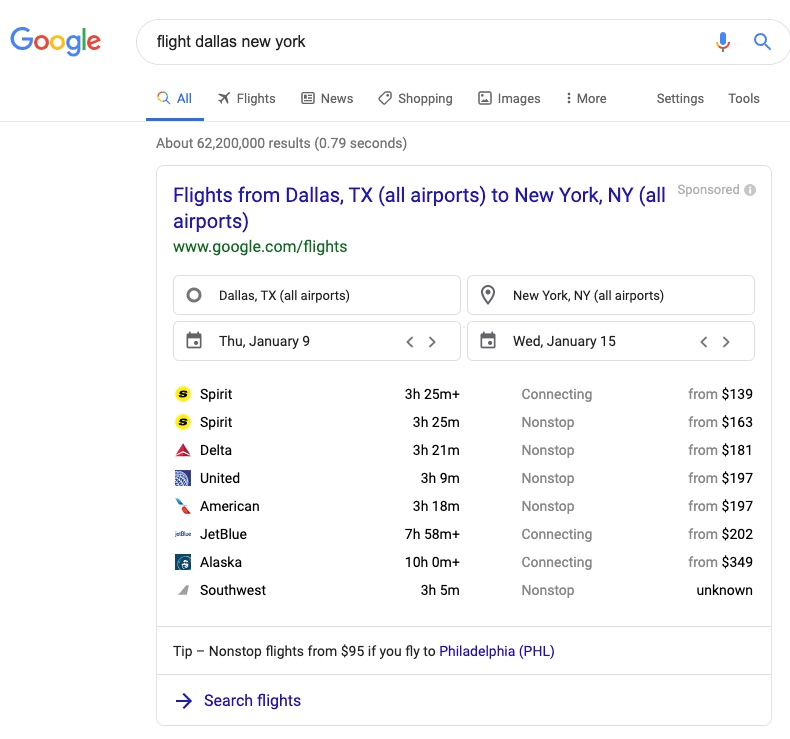A detailed and descriptive caption for the image would be:

"A screenshot of a Google search results page is prominently displayed. At the top, the iconic Google logo is visible in its vibrant blue, red, yellow, and green colors. The search query 'flight status, or flight Dallas, New York' is entered in the search bar, which includes the Google microphone icon and the search magnifying glass. The 'All' tab is highlighted in blue, consistent with Google's traditional color scheme. Other available tabs include Flights, News, Shopping, Images, along with options for more settings and tools.

The search results indicate approximately 62,200,000 results rendered in 0.79 seconds. The first result is a sponsored link in blue text, 'flights from Dallas, Texas (All Airports) to New York, New York (All Airports),' followed by the URL 'www.google.com/flights' in green text. Further down, there are options specified in green hyperlink text for flights from Dallas, Texas to New York, leaving on Thursday, January 9th and returning on Wednesday, January 15th. Various airlines such as Spirit, Delta, United, and American are listed as options for these routes."